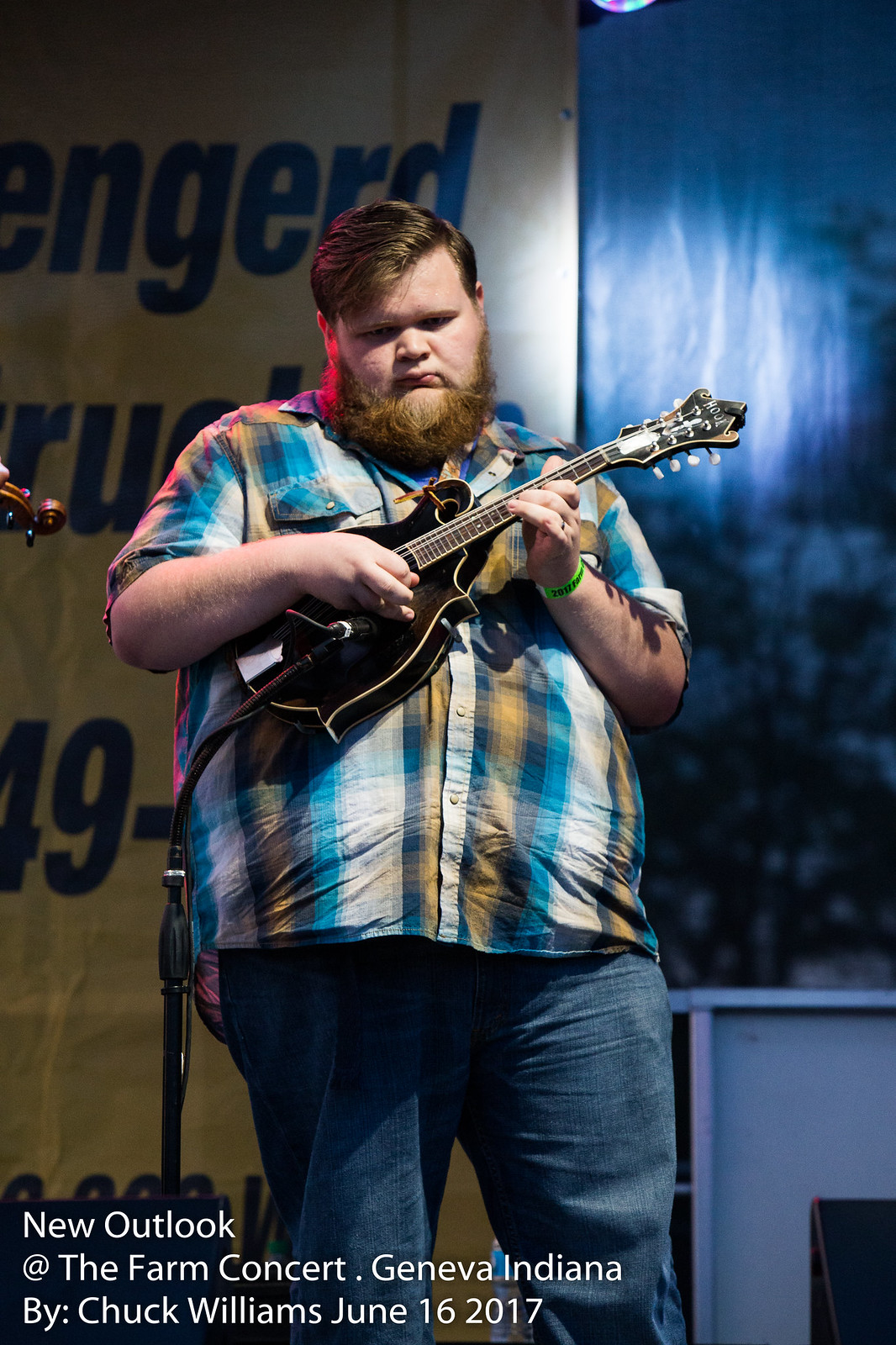In this image, a large Caucasian man with pale skin, who appears mildly overweight, is captured on stage. He sports a short-sleeve, button-down plaid shirt with blue, yellow, and white patterns, and he pairs this with blue jeans. A green wristband adorns his wrist. His hair is a mix of brown and blonde, and he has a similarly colored beard. He is playing a small string instrument that resembles a ukulele or a modern-looking banjo, and there is a microphone positioned in front of him. An electric cord is attached to his instrument, suggesting it's electric. The backdrop features a large, partially visible sign in blue and yellow with illegible text. The bottom left corner of the image contains white sans-serif text that reads, "New Outlook at the Farm Concert, Geneva, Indiana, by Chuck Williams, June 16, 2017." The setting of the performance, whether indoor or outdoor, is not clear.